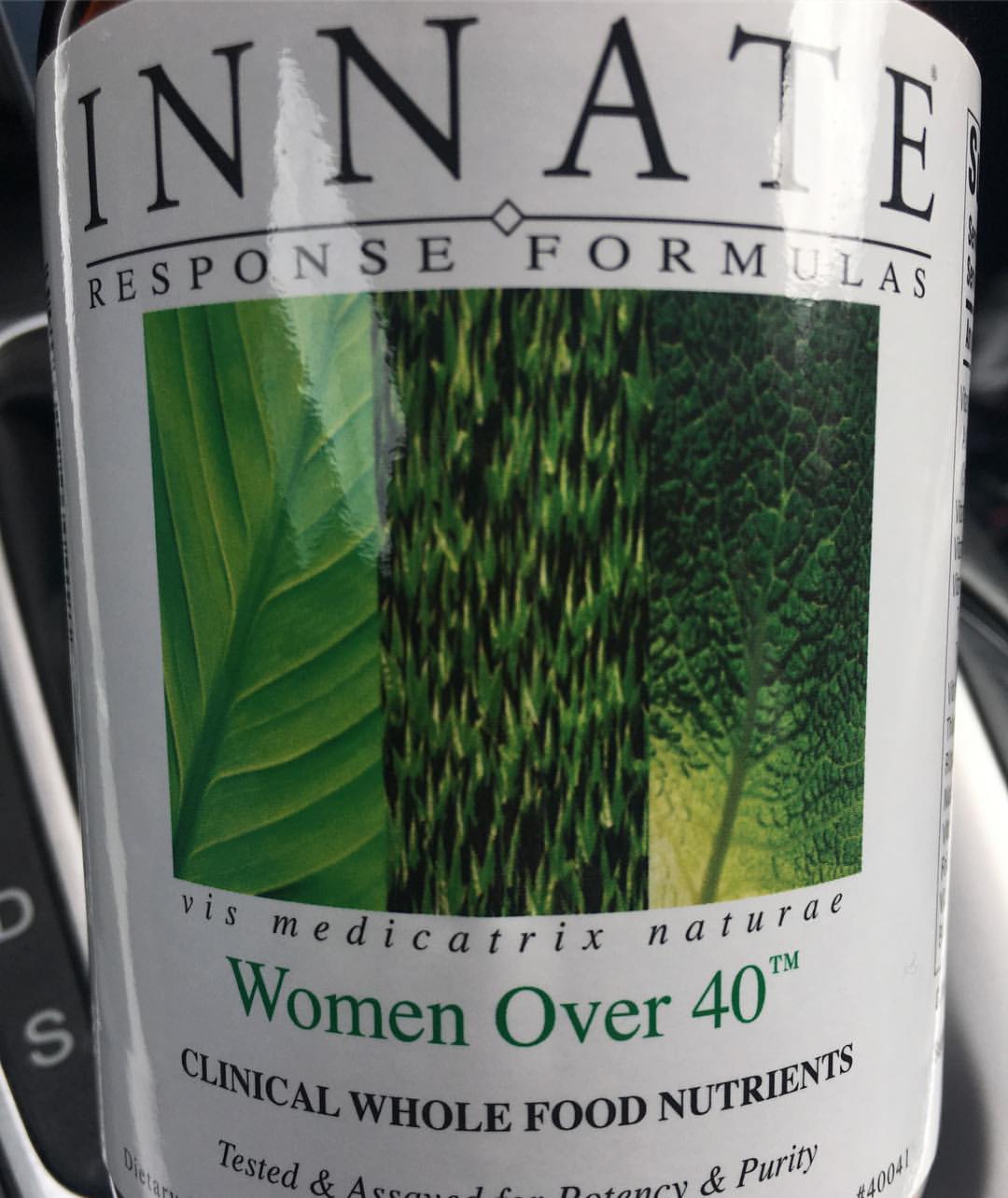The image is an extreme close-up, indoor color photograph of a product label on a cylindrical object, possibly a supplement container. The label has a white background. At the top, in black capital letters, it says "INNATE," followed by a horizontal black line, and below it, in smaller black capital letters, it reads "RESPONSE FORMULAS." There is a square image displaying a close-up of three green leaves, showcasing their patterns with the middle one resembling grass. Below the image, in black capital letters, it says "VIS MEDICATRIX NATURAE." Underneath, in green font with a superscript "TM," it reads "WOMEN OVER 40." Further down in black capital letters and a smaller font size, it states "CLINICAL WHOLE FOOD NUTRIENTS." The phrase "tested" appears partially visible towards the bottom, cut off by the image's lower edge, and then continues with "and purity." The top and bottom of the cylindrical object are not visible in the image.